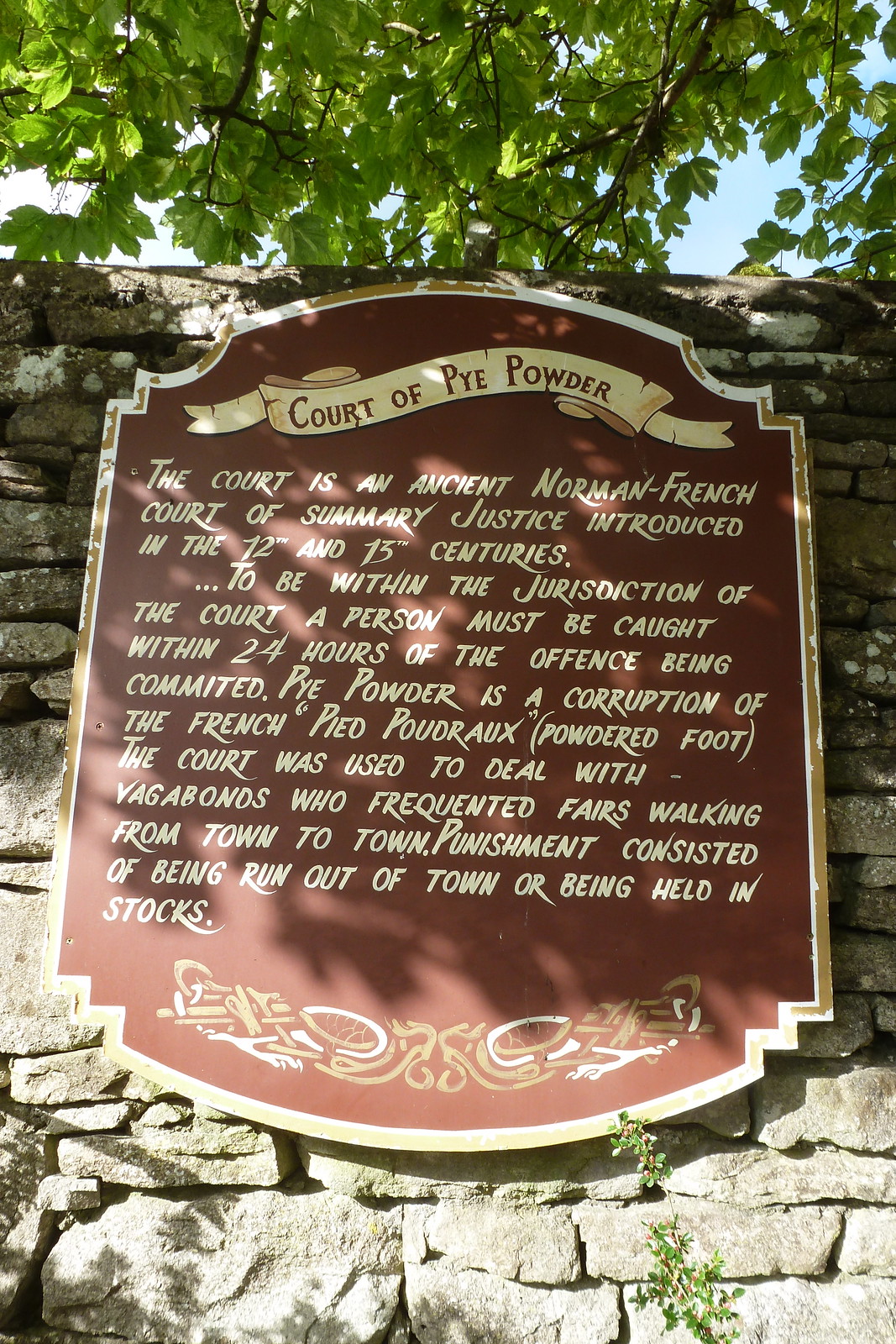The image depicts a detailed outdoor plaque mounted on a diverse-sized stone wall with a few green tree leaves visible above. The plaque is crafted in a square shape with rounded corners and features arch designs at the top and bottom. At the top, a painted banner reads "Court of Pied Powder." Below, the text narrates the historical significance of this Norman French court of summary justice, introduced during the 12th and 13th centuries. According to the inscription, the court dealt with offenders, specifically vagabonds who frequented fairs, and required that individuals be caught within 24 hours of committing an offense to be within its jurisdiction. The term "Pied Powder" is explained as a corruption of the French "pied poudre," meaning "powdered foot." Punishments meted out by this court included being run out of town or confined in stocks. The text is painted in white on a light brown background, adorned with some decorative elements at the bottom. The sign, which appears to be wooden with a historical design, is securely affixed to a weathered grey stone wall.